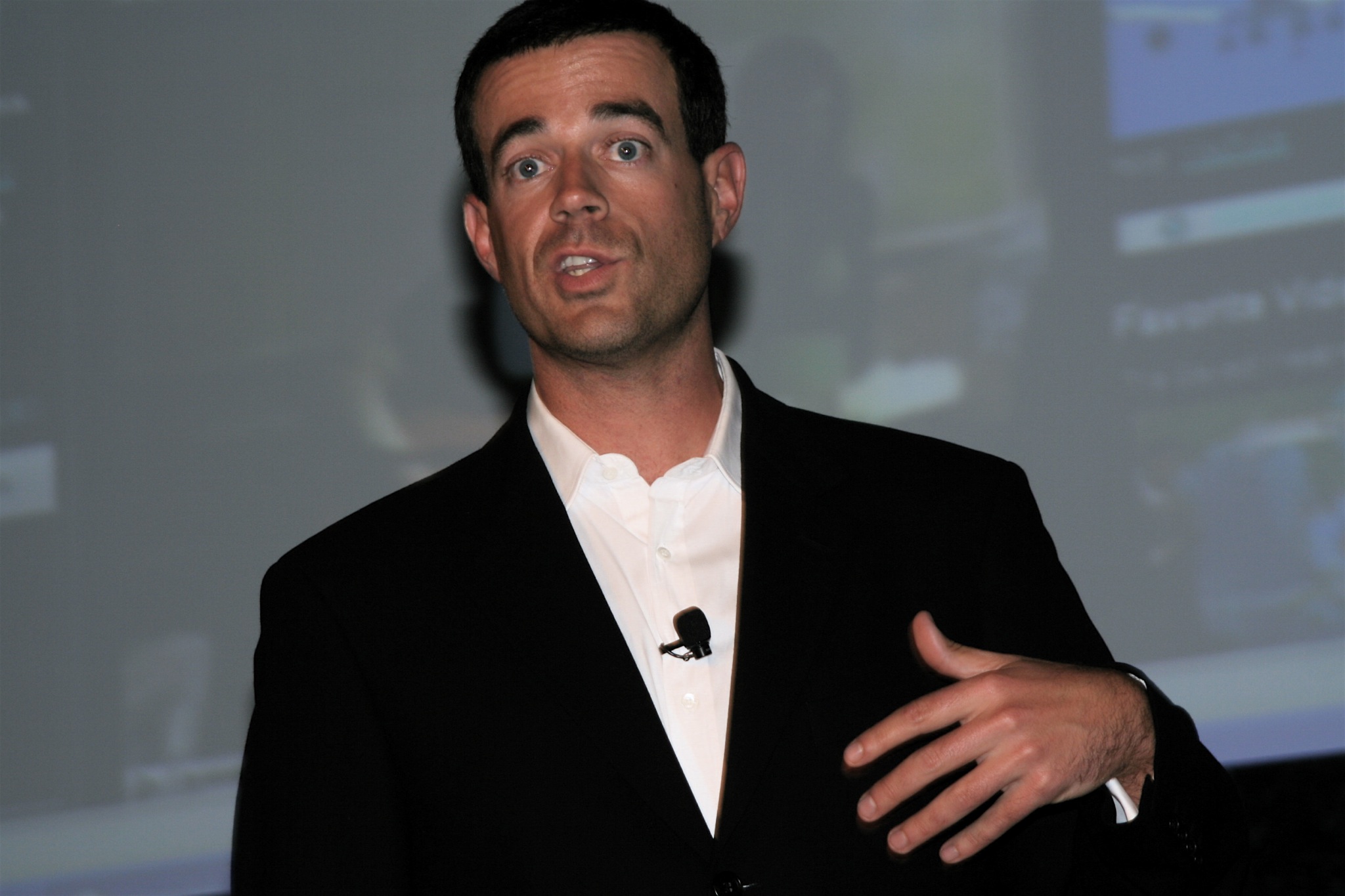The photograph captures a possibly Caucasian man, approximately 30 years old, mid-speech as he gestures with his left hand to emphasize his point. With blue eyes and short black hair that is neatly sculpted, he sports a slight 5 o'clock shadow and a very short mustache. The man is dressed in a black business coat over a white button-up shirt, with the collar's top button undone. A small black microphone is clipped to his shirt, near his chest. His left arm is bent at the elbow, thumb slightly up, and his right arm is out of the frame. Behind him, a blurry projection screen dominates the background, displaying indistinct images of people. The backdrop features a mix of gray, white, and black tones, with some areas of colored light reflections adding further depth. In the lower right corner, a pure black section contrasts with the other elements. The photograph is horizontally aligned and rectangular in shape, capturing the upper part of the man’s body from just below the chest upward.